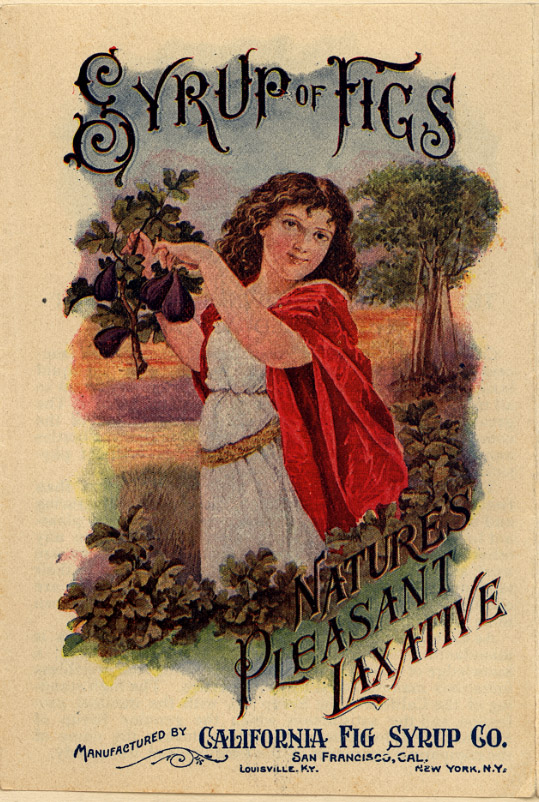This vintage advertisement for the California Fig Syrup Company, with manufacturing locations in San Francisco, Louisville, and New York, showcases their product, "Syrup of Figs, Nature’s Pleasant Laxative." The illustration features a young woman with dark brown, wavy hair, dressed in a classical, Romanesque white dress cinched with a golden belt, and draped in a red cape. She stands amidst fig trees, holding a branch adorned with at least four dark purple figs. The woman gazes off to the right with a slight smile, reminiscent of the Mona Lisa. The background reveals more trees and a scenic sky. The caption emphasizes the natural and gentle essence of the laxative, making it an appealing choice for health-conscious consumers of the time.